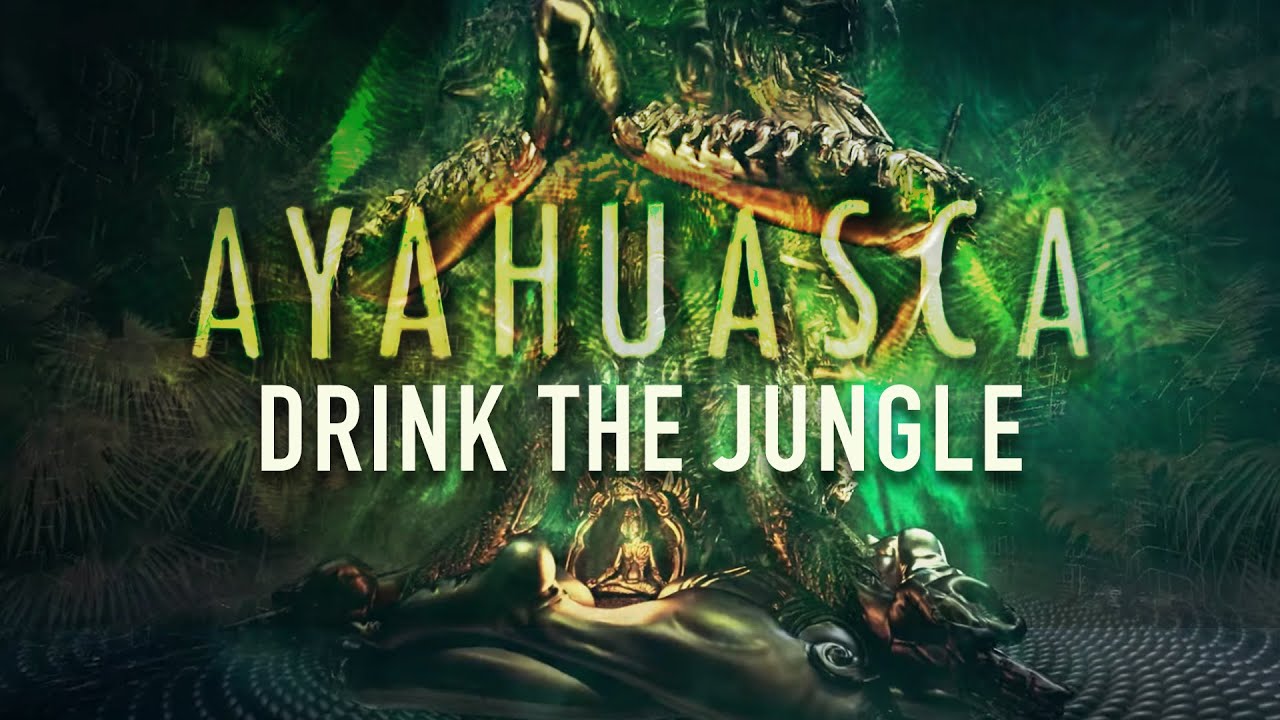This horizontally oriented advertisement resembles a movie or game poster dominated by diverse shades of green. In the center of the image, the word "Ayahuasca" is embossed in prominent green lettering, with the phrase "Drink the Jungle" in white situated just below. Above "Ayahuasca," there's a large, abstract creature that looks like a locust with green scales, prominently featuring a bent leg similar to a frog's, set against a backdrop of lush green palm leaves. Beneath the words "the jungle," within a circular gold frame, a small figure is depicted in a lotus position, seemingly meditating inside a hollowed-out tree. The image background transitions from dark green on the left to lighter shades on the right, heavily adorned with varying green palm leaves and shadows, adding to the mystical jungle ambiance.